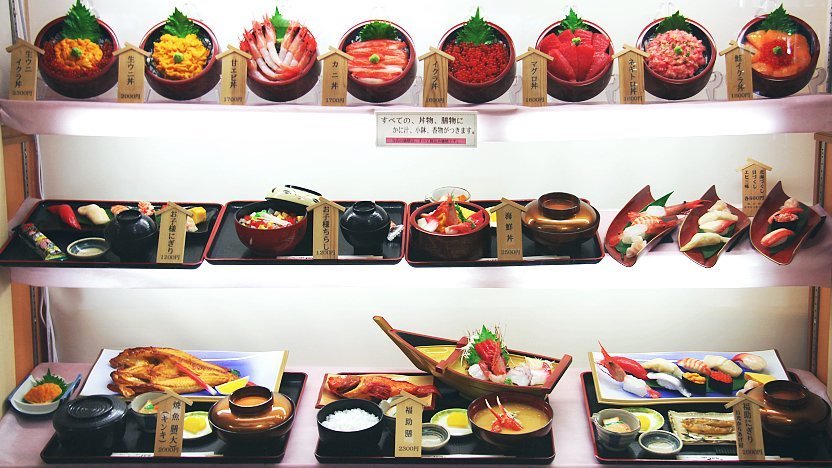The vibrant and colorful photograph showcases a food display set against a white wall, resembling a restaurant setup often found in Japan. It features three shelves adorned with an assortment of detailed and meticulously arranged dishes. The top shelf holds eight round bowls, each facing upwards, revealing a variety of seafood and sashimi. Accompanying the bowls are small wooden labels shaped like birdhouses, inscribed with text in Japanese. The middle shelf includes three black cafeteria trays, each containing neatly labeled meals. To the right of these trays are three additional platters, also laden with seafood. The bottom shelf appears to display the most luxurious and elaborate meals. Large trays filled with abundant portions of seafood and other dishes dominate this shelf. Notably, one tray even features a sushi boat, while another offers what appears to be an array of succulent chicken, complemented by sides of rice. This elaborate setup captures the essence of traditional Japanese cuisine, emphasizing its diversity, richness, and intricate presentation.